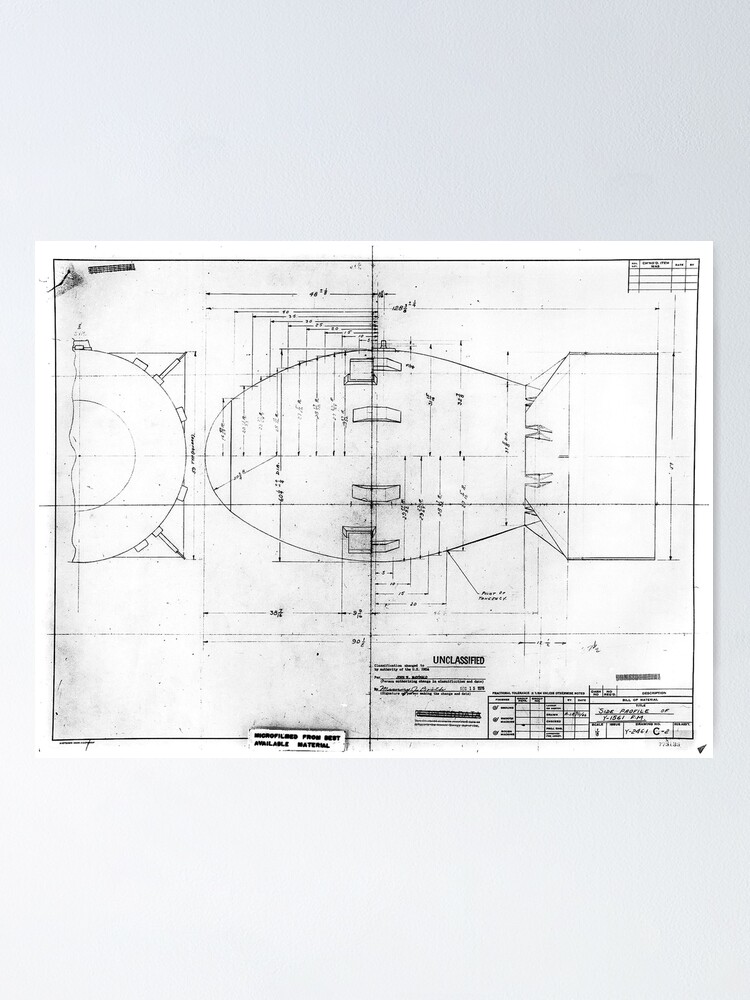The image depicts an aged white paper fixed on a surface transitioning from gray at the top to white at the bottom, showcasing an intricate, black-ink blueprint. The illustration resembles a bomb or rocket, oriented with the front facing left and the back to the right, delineated by multiple lines, numbers, and letters presumably indicating measurements. The design, detailed with a semicircle on the left and an oval-rectangle composite on the right, is surrounded by a thin black border and central dividing line. Despite noticeable smudging, the blueprint includes substantial annotations, although most text is too small to decipher. However, the word "unclassified" stands out at the bottom, accompanied by a chart with various boxes, letters, and numbers. There is also a black-ink block slightly left of center, further contributing to the comprehensive technical layout.